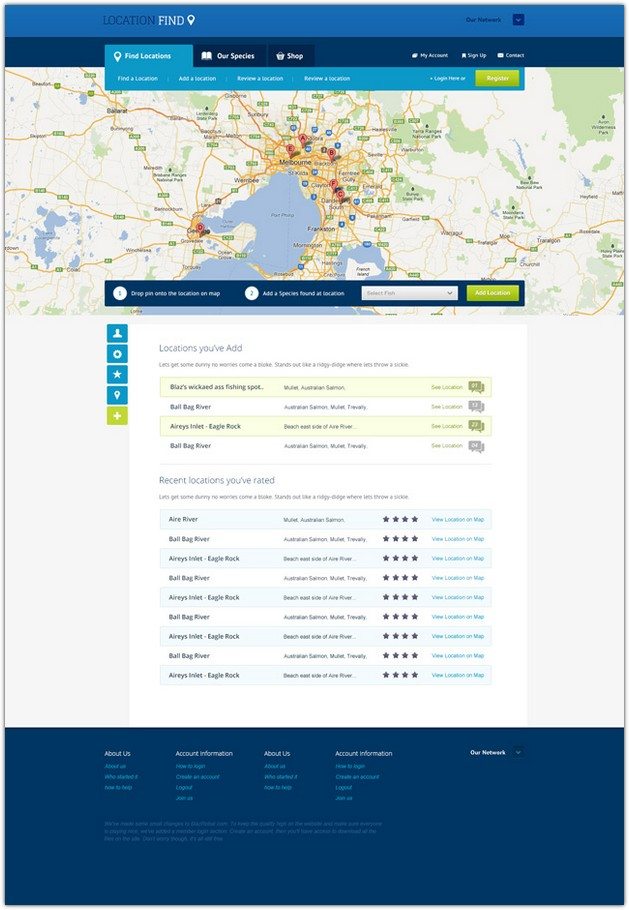This image is a screenshot of a webpage featuring a navigation and location search interface. At the top of the screenshot, there is a blue header with darker blue text that reads "Location," and to its left, there is white text that says "Find." Directly below the header, there is a slightly blurry light blue pull-down menu for finding locations, with options listed as "Find a location," "Add a location," and "Review a location." To the right of the pull-down menu, there is a prominent green button labeled "Register."

Taking up most of the central area of the page is a large map depicting various regions in shades of green, ivory, and red, with a specific emphasis on the area around Melbourne. Finally, at the bottom of the webpage, the footer contains links that are repeated twice: "About Us," and "Account Information." To the right of these links, there is a button with white text that reads "Our Network."